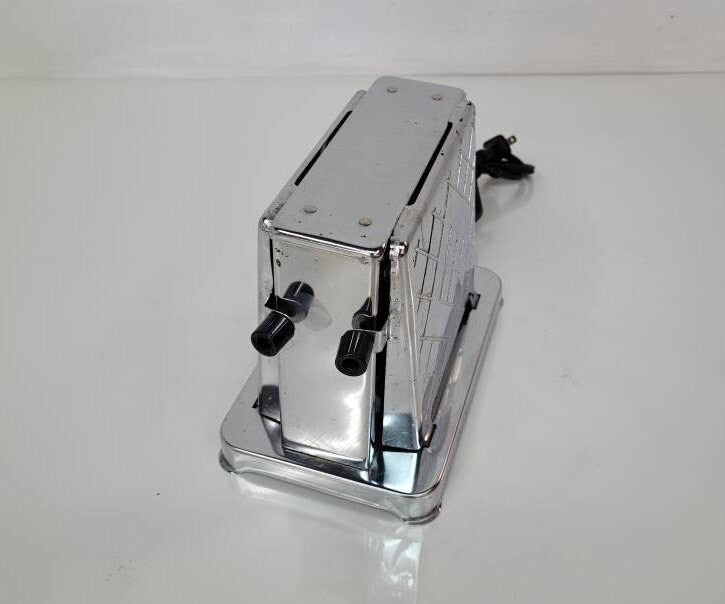This image features a detailed view of a vintage stainless steel appliance, most accurately described as a toaster, positioned on a solid white stone tabletop with a white background. The device, unmistakably crafted from silvery chrome, has a reflective surface that mirrors part of its structure onto the table beneath it. The appliance is designed with a square top and a slightly wider rectangular base. Prominent on its front are two black knobs, appearing to either pull out or lift up the front panel, which showcases a diagonal crisscross design. Behind the appliance, a black cord, likely for plugging in the device, extends towards the back. The top of the toaster seems to have a hinged compartment, hinting at a functional design that deviates from conventional top-slot toasters, suggesting a unique vintage mechanism where the front panel possibly folds down to accommodate whatever it is intended to toast.